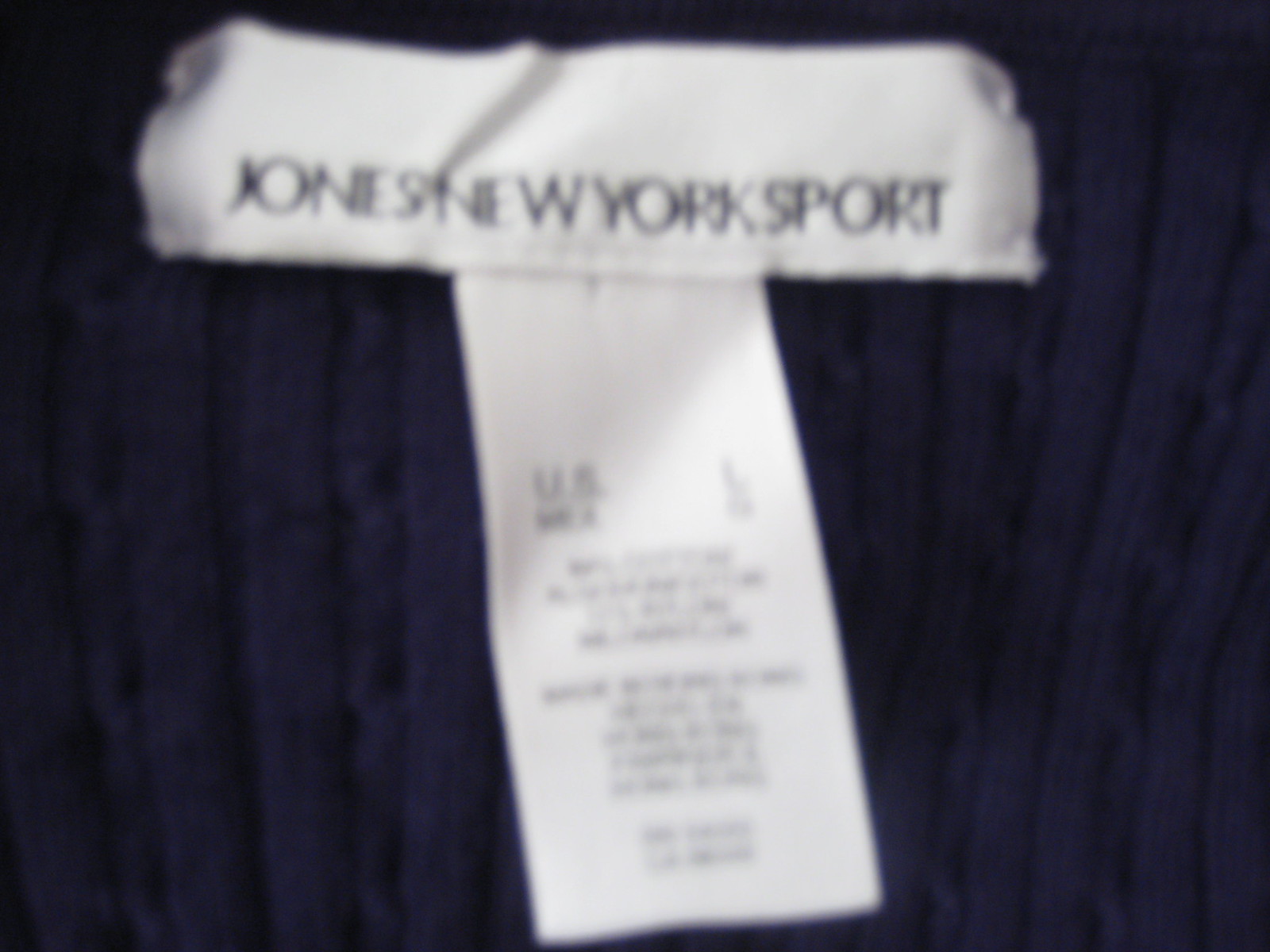This image is a close-up shot of the tag inside a medium to dark navy blue women's cable knit sweater. The sweater's knit structure and fabric density are visible, showcasing the detailed threading. The main white silky tag is prominently displayed and reads "Jones New York Sport" in clear black lettering. Below this, a secondary tag, narrower and also white, is sewn on and appears to contain care instructions, though it’s mostly illegible due to the blurry focus of the image. Only parts of the text, such as "US" in the upper left corner, are faintly discernible. The tag is likely located at the neckline of the sweater, which features vertically knitted cables.